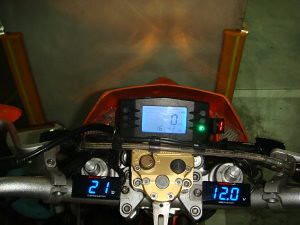This photograph captures the control panel of a motorcycle, focusing on its intricate details. Dominating the panel are three distinct display screens. The central display, partially obscured by a light, shows a digit '0'. Adjacent to it, a green indicator light is visible, set against a black background. Surrounding the controls is a red housing, adding a bold contrast to the setup. At the top of the panel, what appears to be orange handles or mounts likely support a visor or windscreen. Below the central screen, two additional displays are clearly visible, reading '21' and '12.0' respectively. Flanking these displays are dark silver or dark gray handlebars, framing the metal components of the control panel. In the distance, faint brake lights of another vehicle can be seen, suggesting a few car lengths' separation. Additionally, a road marking, possibly a crosswalk line, stretches across the street ahead, indicating that the motorcycle might be stopped at an intersection or pedestrian crossing.